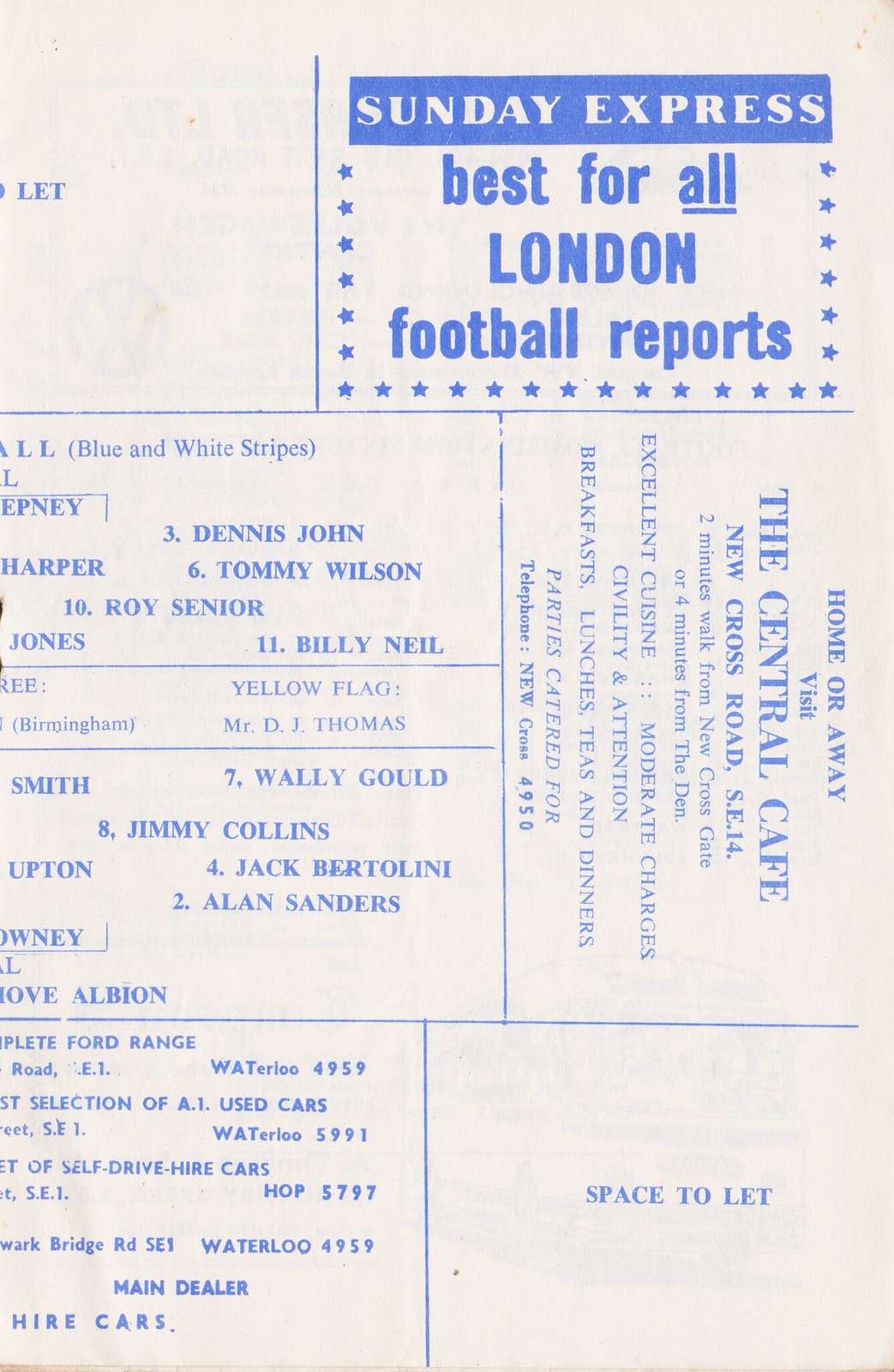The image features an aged piece of paper, possibly a page from an old magazine or newspaper, showcasing promotional material. Dominating the top section is a blue square with white text reading "Sunday Express," followed by the phrase "Best for All London Football Reports," adorned with small stars. The background of the paper is a yellowed, off-white color.

The left side of the document is occupied by a large list of football players, including names and numbers such as:
- Number 3: Dennis John Harper
- Number 6: Tommy Wilson
- Number 7: Wally Gould
- Number 8: Jimmy Collins
- Number 10: Roy Senior Jones
- Number 11: Billy Nail
- Number 4: Jack Bertolini
- Number 2: Alan Sanders
- Number ??oni (partial, cut off)
- Yellow flag: Mr. J.D. Thomas

An advertisement on the right, printed sideways, promotes the "Central Cafe" located at New Crossroads SE14, emphasizing its proximity to local landmarks and public transport options. It highlights offerings such as breakfast, lunches, teas, dinners, and party catering services, with the phone number "New Cross 4950" provided for inquiries. A smaller section below mentions "space to let."

The layout is scattered and text appears in various orientations, giving it a disorganized yet historically rich feel. The overall appearance and content suggest it is a vintage sports-related document, providing a glimpse into both football reporting and local business promotion from a bygone era.